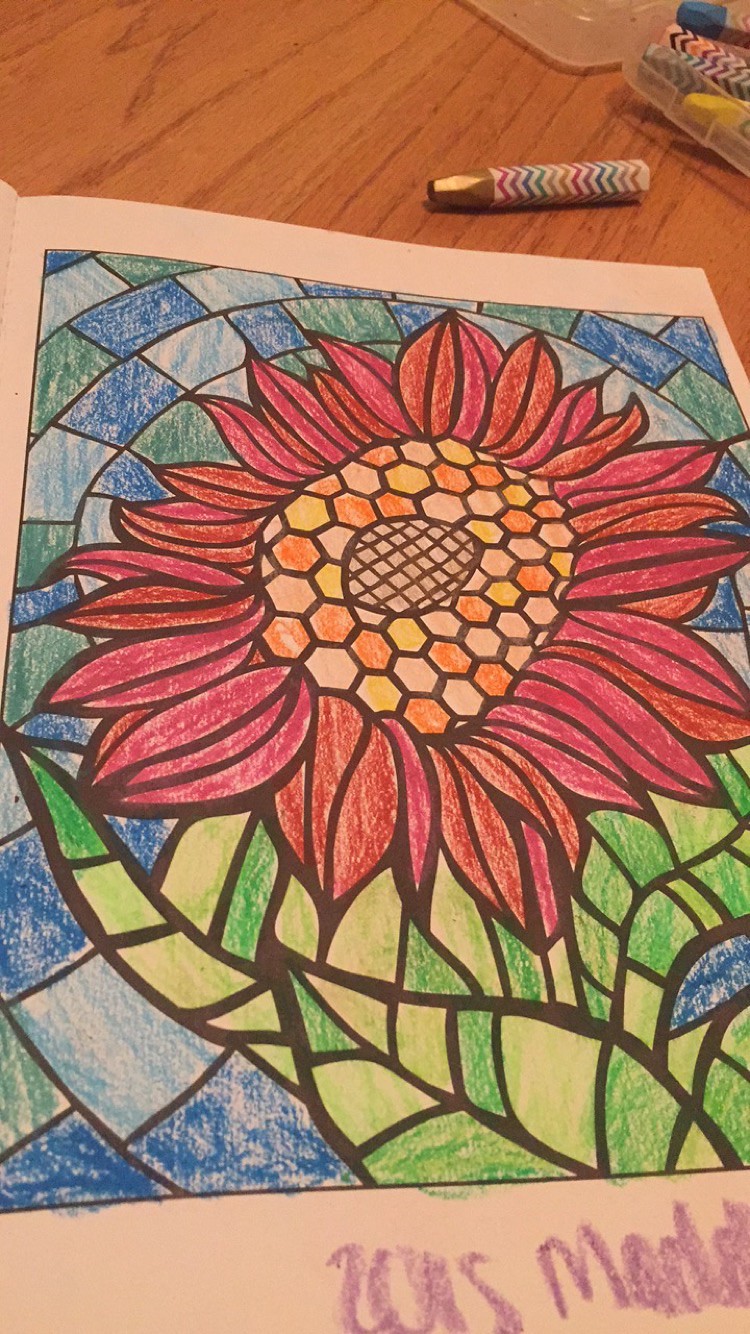The image portrays a meticulously colored page from a coloring book. The book lies open to a white page bordered by a thin black line, typical of many coloring books. Dominating the page is a vibrant flower with red petals, shaded with hues of orange-red and brownish-red. The petals are relatively short, featuring a wavy and sharp design, encircling a large, intricate center. The flower's center is designed with honeycomb-shaped boxes outlined in black, filled with shades of orange, peach, and yellow. Within this central area is a donut-shaped pattern composed of a mesh of black lines interspersed with the white of the page.

Surrounding the flower are green leaves and blue boxes arranged in a circular stone-like pattern, adding an element of depth and structure to the artwork. The entire scene is set against a light wooden surface, showcasing a natural brown color with darker brown grain patterns. Resting beside the coloring book is a crayon, marked by a white label adorned with multicolored lines - reds, greens, blues, yellows, and browns - against a backdrop of gold. This crayon, positioned on the wood, hints at the creative process behind the beautifully colored illustration.